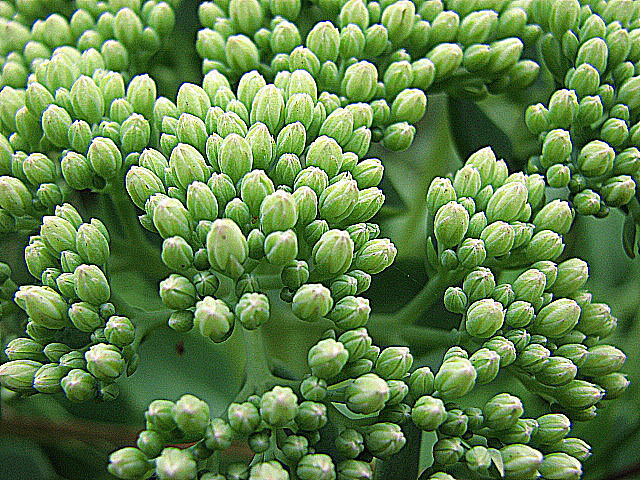The photo is a detailed close-up of a plant viewed from above, focusing on clusters of small, compact buds or flowers. The buds are tightly packed together, forming larger conical or rounded structures branching off from central stems. Each bud is a vivid, leafy green with hints of white, and a few show a slight opening at the top, revealing the possibility of pink flowers inside. The texture of the buds is fleshy and succulent, suggesting a plant adapted to conserve moisture. The arrangement of the clusters exhibits a fractal-like pattern, with repeated smaller subunits. The central part of the plant is in sharp focus, displaying its lush, healthy green color, while the surrounding buds blur toward the edges of the frame, enhancing the depth of the image. The background is a blurred green, likely the leaves, providing a soft contrast to the detailed buds. The entire scene captures the plant's vigorous early blooming stage, with all buds in a nearly identical state of opening.